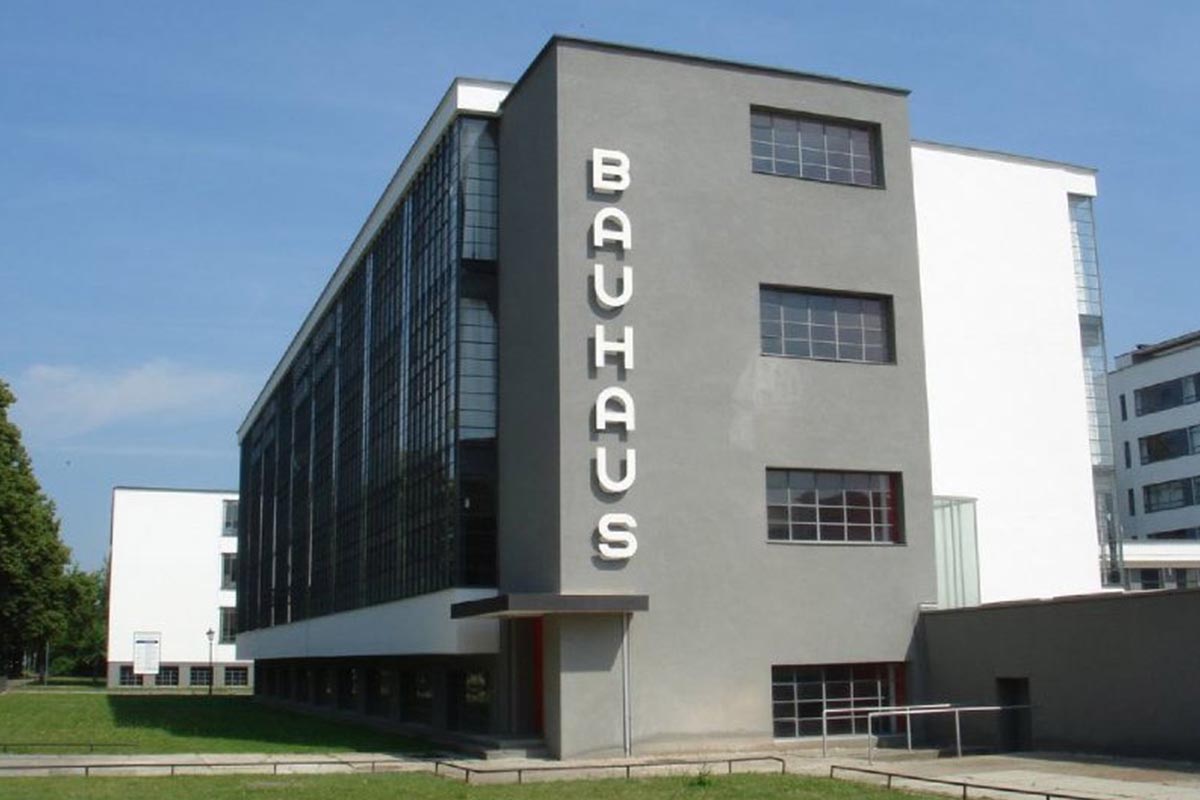The image captures a striking view of a multi-story Bauhaus building under a bright blue sky with a small white cloud on the left. The building, positioned centrally in the photo, features a prominent grey wall with the word "B-A-U-H-A-U-S" engraved in large white letters, vertically aligned from top to bottom. This grey facade also includes four big rectangular windows arranged in a vertical row on the right side of the wall. The left section of the building's profile shows a white roof and a black outer wall, with the top of the ground floor also painted white. The front of the building, viewed from a side angle, is largely made of glass. In front of the building stretches a lush, green field of grass, and to the left, more grass leads up to a scene of trees. To the right of the building, a short wall extends toward the camera, with stairs leading down to an entrance. Additionally, behind and to the right of the Bauhaus structure, other buildings and trees are partially visible.